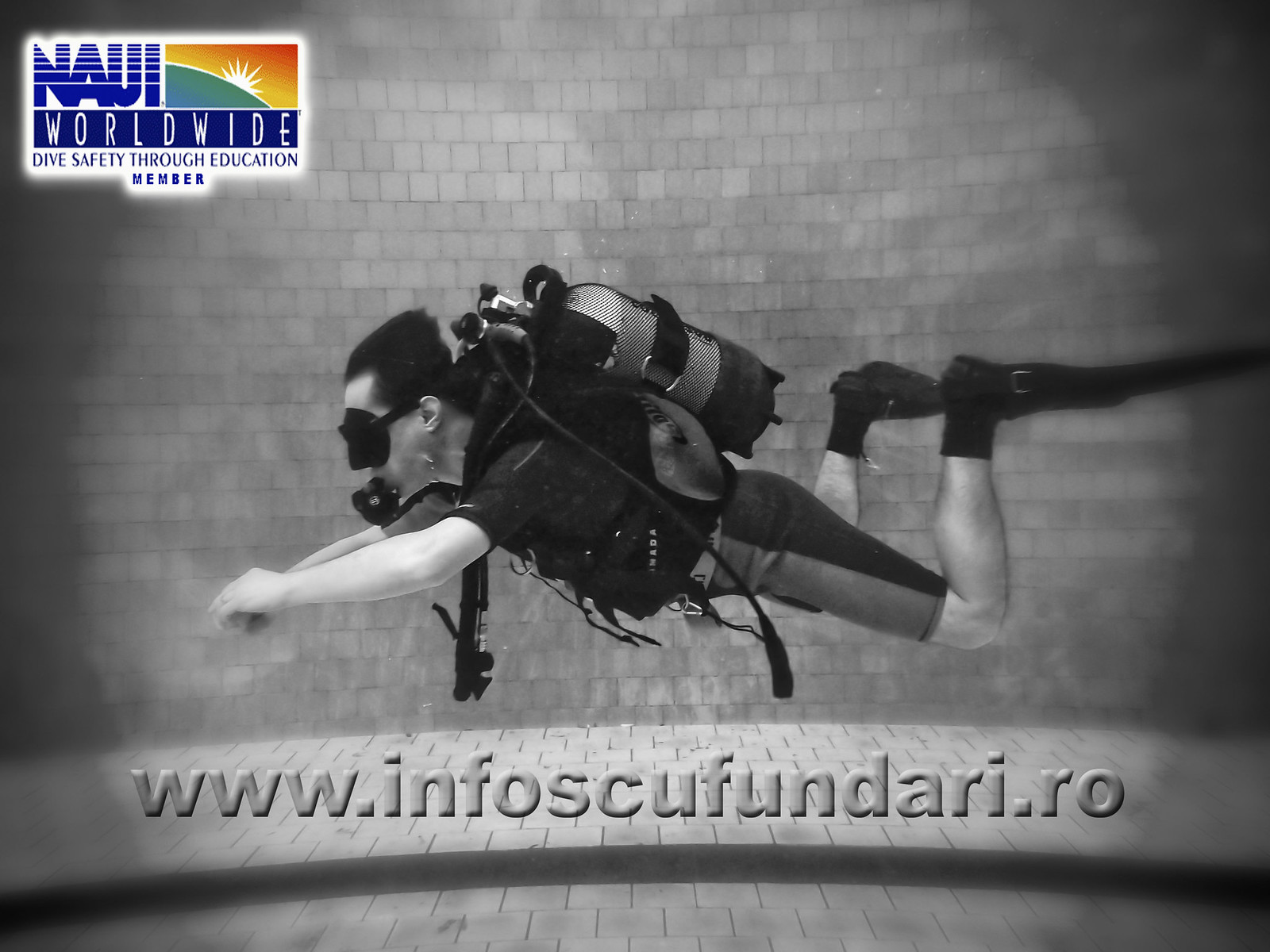The image features a striking advertisement for NAUI Worldwide's Dive Safety Through Education program. Positioned against a textured brick or tile wall, a scuba diver fully equipped with modern scuba gear, including a tank and face mask, appears to be suspended mid-dive in a pool. The diver's horizontal pose, with arms outstretched and knees slightly bent, adds a dynamic element to the image. In the upper left corner, the NAUI Worldwide logo is prominently displayed, featuring the tagline "Dive Safety Through Education" above the word "member," accompanied by a vibrant depiction of a globe with the sun rising behind it. At the bottom of the image, the URL www.infoscufundare.ro is clearly visible, directing viewers to more information about diving safety and courses offered by the organization. This visually captivating ad serves as a powerful reminder of the emphasis NAUI Worldwide places on dive safety and education.